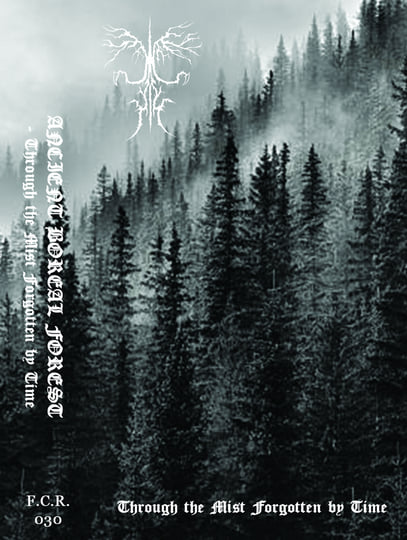In this black and white photograph, a mist-covered forest stretches across a hillside thick with tall, dark pine trees. The mist weaves through the dense foliage, creating an ethereal and timeless atmosphere. At the bottom left corner in small, white text, the initials "F.C.R" are followed by the number "030." Just to the right of this, in cursive white text, are the words "through the mist forgotten by time." This phrase is repeated twice more: once vertically in an ornate font along the left side of the image accompanied by nearly illegible foreign letters, and again horizontally in the middle left-hand side. In the top left corner, an abstract logo resembling lightning and cloud forms in varying shades of gray adds a mysterious touch. The overall scene conveys a cold, misty setting in an ancient boreal forest, beautifully captured in monochrome.